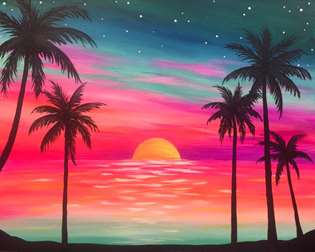This painting depicts a stunning tropical sunset scene with a rich and vibrant palette. The sky is a breathtaking blend of colors, transitioning from deep red and pink near the horizon, through shades of orange, yellow, light blue, to darker blues and purples as it reaches the top. Scattered across this colorful expanse are delicate white stars, adding a touch of magic to the atmosphere. In the center of the sky, the sun, painted in a golden hue, appears to either be setting or rising, casting a warm glow over the scene. Below the sun, a river or body of water mirrors these vivid colors, shifting from orange and white near the horizon to a lighter blue as it reaches the foreground. On either side of the painting, majestic palm trees with black trunks and dark, foliage frame the scene, enhancing its tropical charm. The ground beneath the trees is rendered in solid black, perhaps representing the darkened shore or beach. This captivating artwork beautifully captures the tranquil yet dynamic spirit of a sunset in paradise.